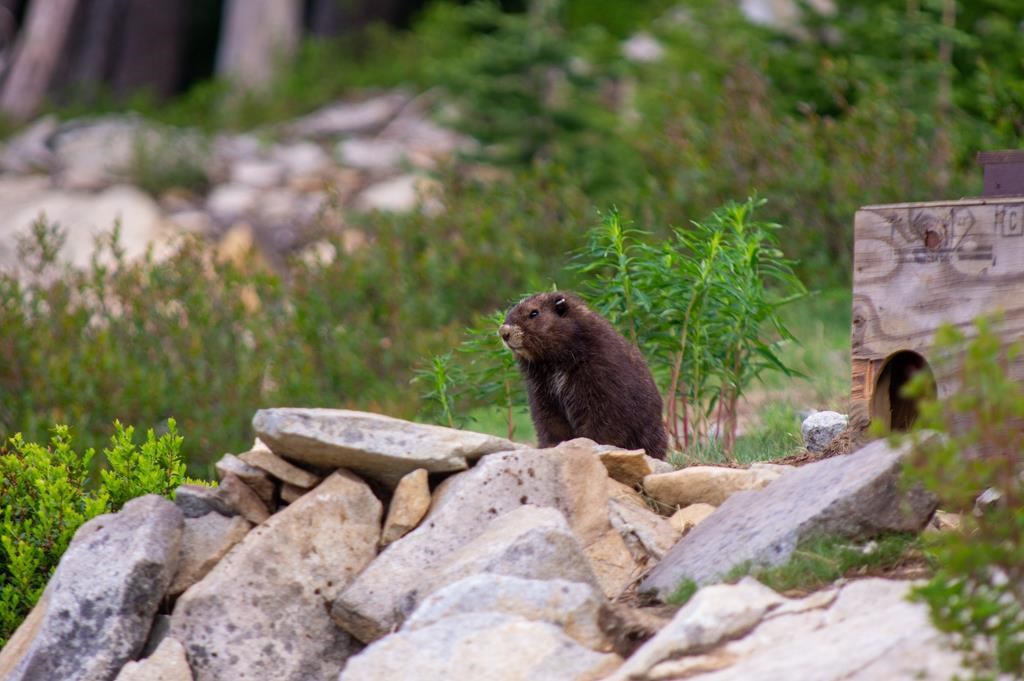This detailed color photograph captures a small rodent, its species uncertain but possibly a chipmunk, beaver, or nutria. The animal has dark brown fur with a light brown snout, white around its nose and mouth, and black eyes. It is emerging from behind a large pile of mostly white and tan rocks accented with black and brown tones. 

Surrounding the rodent are leaves and various shades of green foliage, suggestive of a natural habitat. The background is out of focus but reveals additional leaves, rocks, and tree bark in an array of colors including black, white, gray, tan, brown, and hints of yellow. 

To the right of the image is a man-made wooden crate with a noticeable oval hole, potentially serving as a shelter for the rodent. Despite its natural setting, the photograph appears to have been taken professionally, with the rodent as the main subject. There is no visible text in the image.